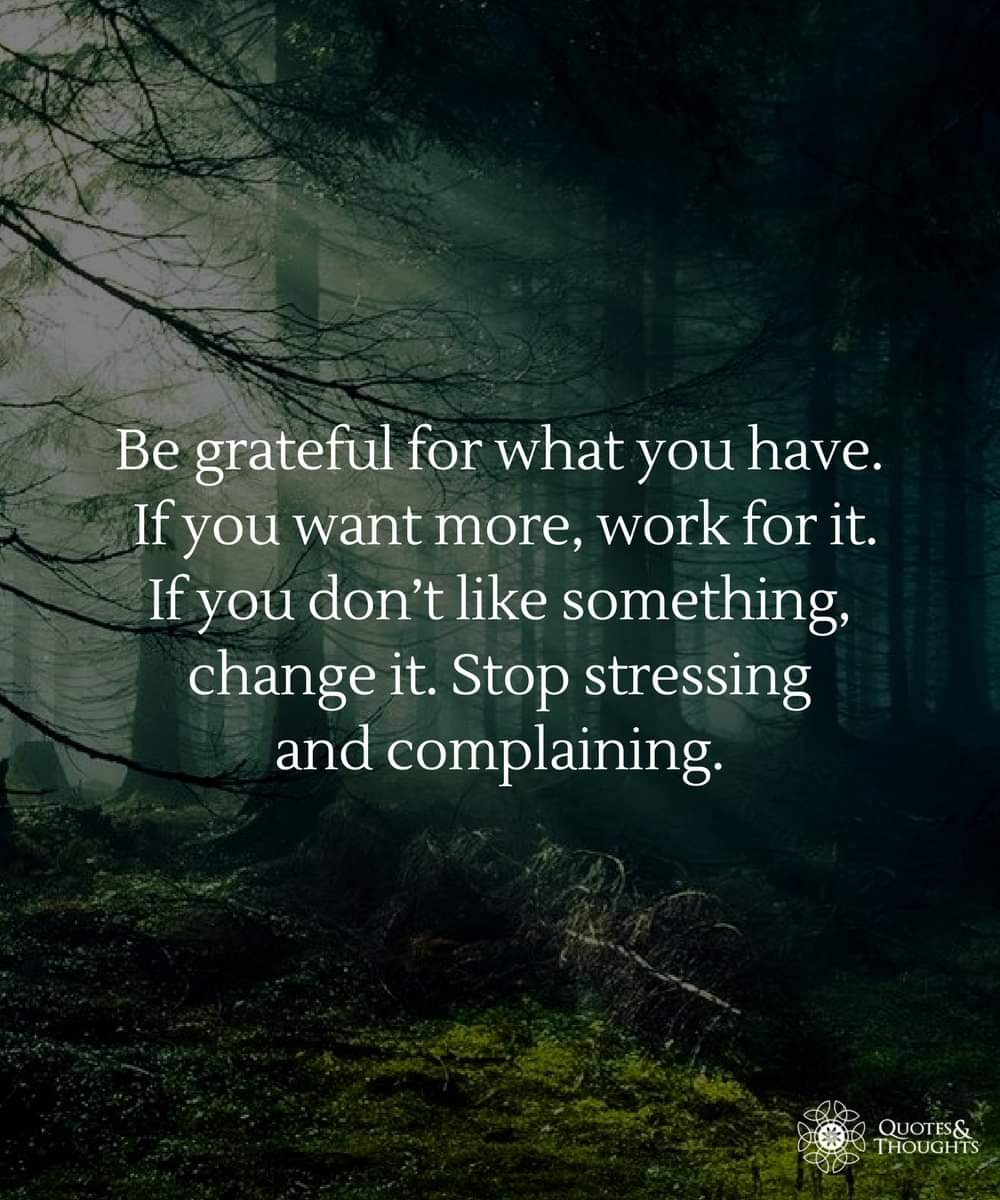This poster features a dark, shadowy forest scene, imbued with green and black tones, complemented by a swirling gray mist. The forest is dense, filled with numerous trees, barren branches, and pine needles. A thin, dry branch lies on the moss-covered ground, adding to the ominous and foreboding atmosphere. There is a slight haze as rays of light peek through on the left side, indicating early morning or a foggy day.

Superimposed on this moody backdrop is an inspirational quote in white lettering, prominently placed in the center of the poster. The quote reads, "Be grateful for what you have. If you want more, work for it. If you don't like something, change it. Stop stressing and complaining." This motivational message stands out clearly against the dark background.

In the bottom right corner, also in white text, is a spiral-like logo accompanied by the words "Quotes and Thoughts," providing a subtle watermark that ties the poster's theme together. The overall composition creates a strong visual and emotional impact, merging the eerie beauty of the forest with uplifting advice.